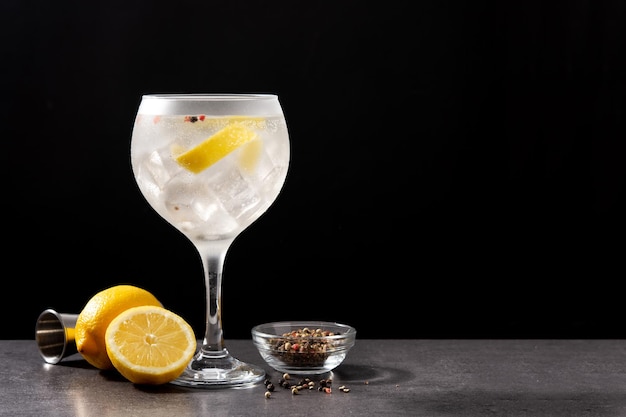This image captures an elegant still life against a dramatic black background atop a sleek, stone countertop. At the forefront stands a frosted, translucent goblet, resembling a large wine glass, filled with a refreshing blend of ice water, lemon slices, and a sprinkle of red and purple garnish, possibly peppercorns. To the left of the glass sits a whole lemon and a halved lemon, showcasing its juicy, segmented interior. Behind the lemons, a small, thimble-sized metal cup is subtly placed, possibly used for measuring. In front of the glass, a small glass bowl brims with dark-colored peppercorns, with a few scattered loosely on the surface, adding a rustic touch to the composition. The overall scene evokes a sense of freshness and meticulous detail.